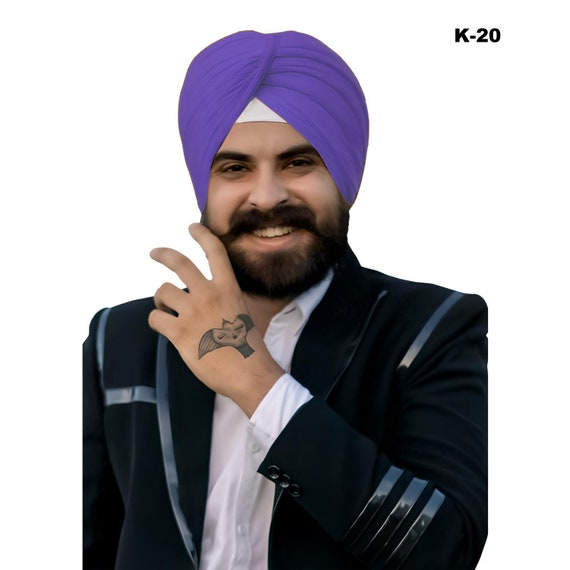This photograph features a man, identified as a sheik, set against a plain white background. In the upper right corner, the image is labeled "K-20." The man has a medium skin tone and is adorned with a well-groomed black beard and mustache. He is smiling, revealing his teeth. He wears a traditional purple turban with a white cap underneath it. His attire includes a black suit jacket with shiny black vinyl stripes - three on the sleeves and a border along the lapel. Underneath the jacket, he dons a white dress shirt. His left arm is raised across his body, partially covering the lower portion of his face and allowing a view of his hand, which bears a tattoo depicting a flying bird with a skull in the middle.